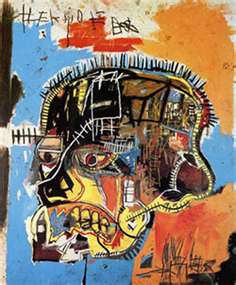This image is an abstract painting reminiscent of Basquiat's semi-graffiti style, characterized by a chaotic and modern aesthetic. Central to the image is a human-like head, potentially representing a skull, with strikingly disordered yellow teeth and spiky hair. The face incorporates various abstract elements and colors, with black overlays and distinct features like eyes, ears, and a mouth. The background is predominantly blue with splotches and scratches of orange, red, yellow, and white, creating a dynamic and destructive appearance. There are illegible writings at the top, and a scribbly black signature is located in the bottom right corner. The composition, taking up about three-fourths of the image, lacks a neck or body, emphasizing the disjointed and fragmented nature of the subject.